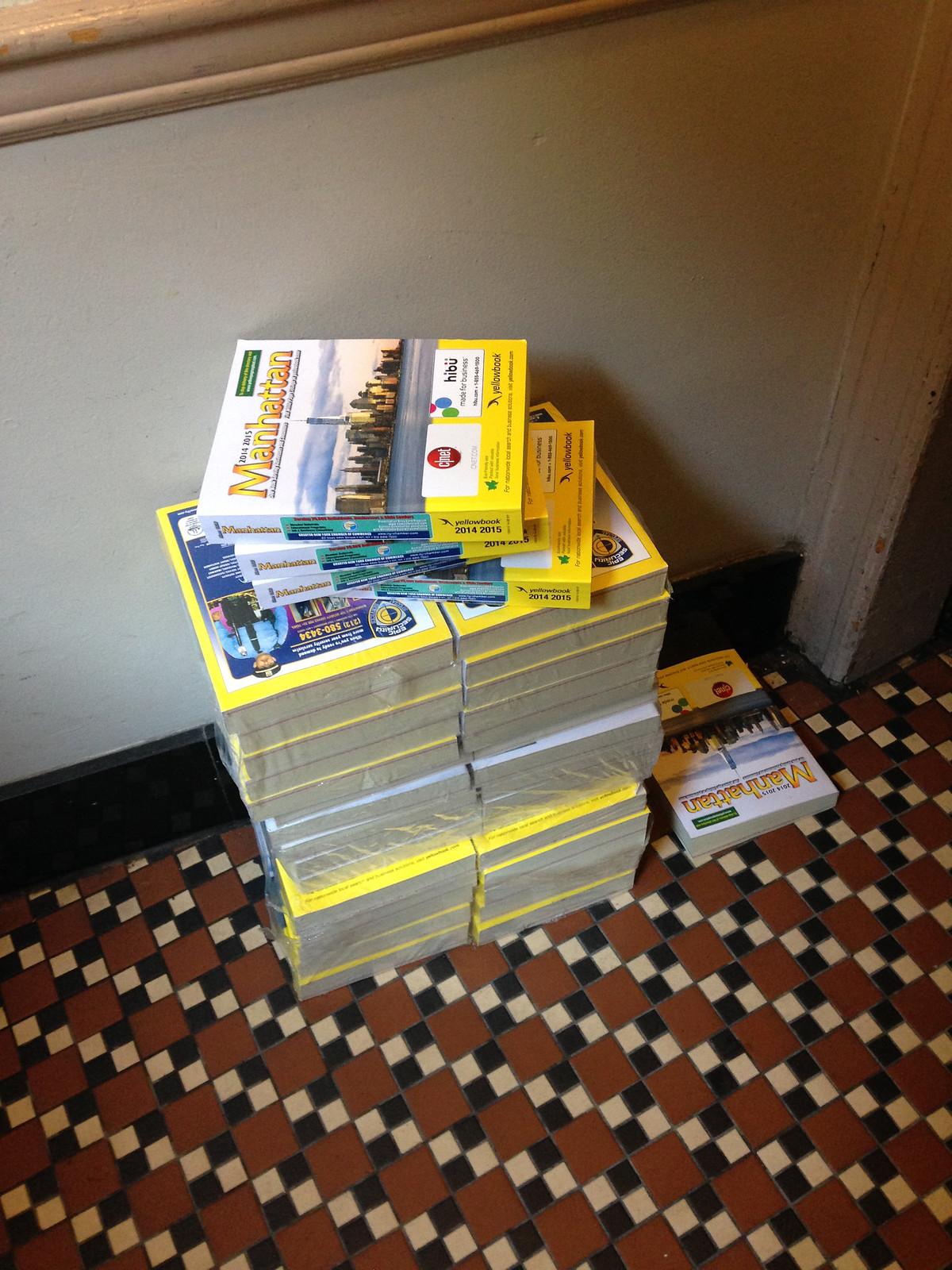The photograph depicts two tall stacks of phone books, each wrapped in plastic, positioned against a gray wall with a thick black baseboard at the bottom. The stacks are situated in a hallway that resembles a commercial building, evident from the door frame visible on the right and a wooden railing or structure at the top edge of the image. Each stack comprises three shrink-wrapped groupings of phone books, with approximately a dozen books per side. Atop these, there are four unwrapped phone books placed unevenly, forming a diagonal. The front cover of the books displays the word "Manhattan" in gold-yellow letters above a photograph of the New York City skyline, prominently featuring the Freedom Tower. A stray notebook lies on the diamond-patterned tiled floor, which alternates between solid dull-red squares and black-and-white checkered squares.